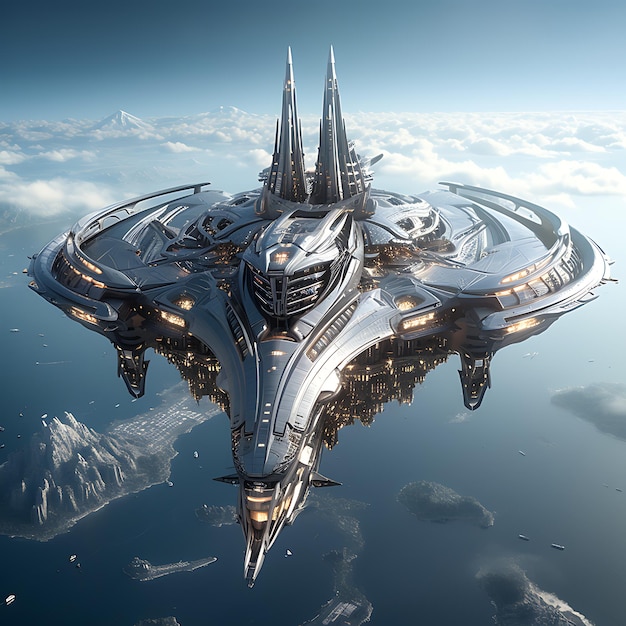This image is a highly detailed, digitally-generated concept art of an ornate, futuristic spaceship soaring above an expansive ocean. The spaceship has a metallic gray and golden hue with a design resembling a blend of the Star Trek Enterprise and a militaristic battleship. It features a roundish main body that extends into a pointed front, evoking a helmet-like visage reminiscent of Transformers or Thanos from Marvel. On its top, two cone-shaped structures protrude like turrets, adding to its imposing and defensive appearance. The spaceship's surface is adorned with numerous tiny windows brightly lit, suggesting a massive interior, almost akin to a flying city. Below, serene, calm water is depicted alongside islands with towering, white mountainous regions. Above the spaceship, a blue sky and a row of clouds frame the scene, enhancing the overall grandiosity and futuristic essence of the artwork. The underside of the ship appears darker and more rugged, contributing to the impression of a heavily-shielded, robust vessel unlike anything seen before.